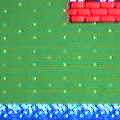The image appears to be a small, square screen from a video game, likely animated in style. Dominating the upper right corner, there are three horizontal rows of bright red bricks, outlined in black. The majority of the background is green with evenly spaced white dots arranged in vertical columns, reminiscent of a farm or field. The bottom portion of the screen transitions from a light blue at the top to a darker shade of blue below, lined with white dots that stretch horizontally. This bottom section might represent a border or part of the game interface. The overall scene and layout suggest it could be from a classic farm-themed arcade game.